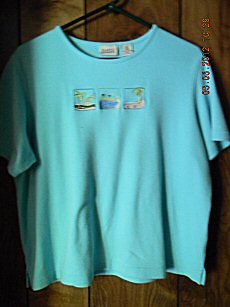This photograph captures a t-shirt hanging on a black hanger against a brown wooden wall. The t-shirt, which is a light teal or baby blue color, features short sleeves and appears slightly wrinkled. On the front chest area, there are three small rectangular graphics. The exact details of these graphics are unclear, but one image seems to depict greenery, the middle graphic might contain a lighter blue object resembling a boat, and the third has pink elements. Additionally, there’s a label in the center of the neckline and another label immediately to its right. On the left sleeve, a series of small reddish numbers appears to be superimposed or Watermarked onto the photograph. The wall exhibits a slight color variation above the left corner, where it's a bit lighter. Shadows accentuate the corners of the photograph and part of the t-shirt's left sleeve. Some text, possibly indicating a date and time, might be positioned in the upper right-hand corner of the image, reminiscent of an old photograph or video recording timestamp.